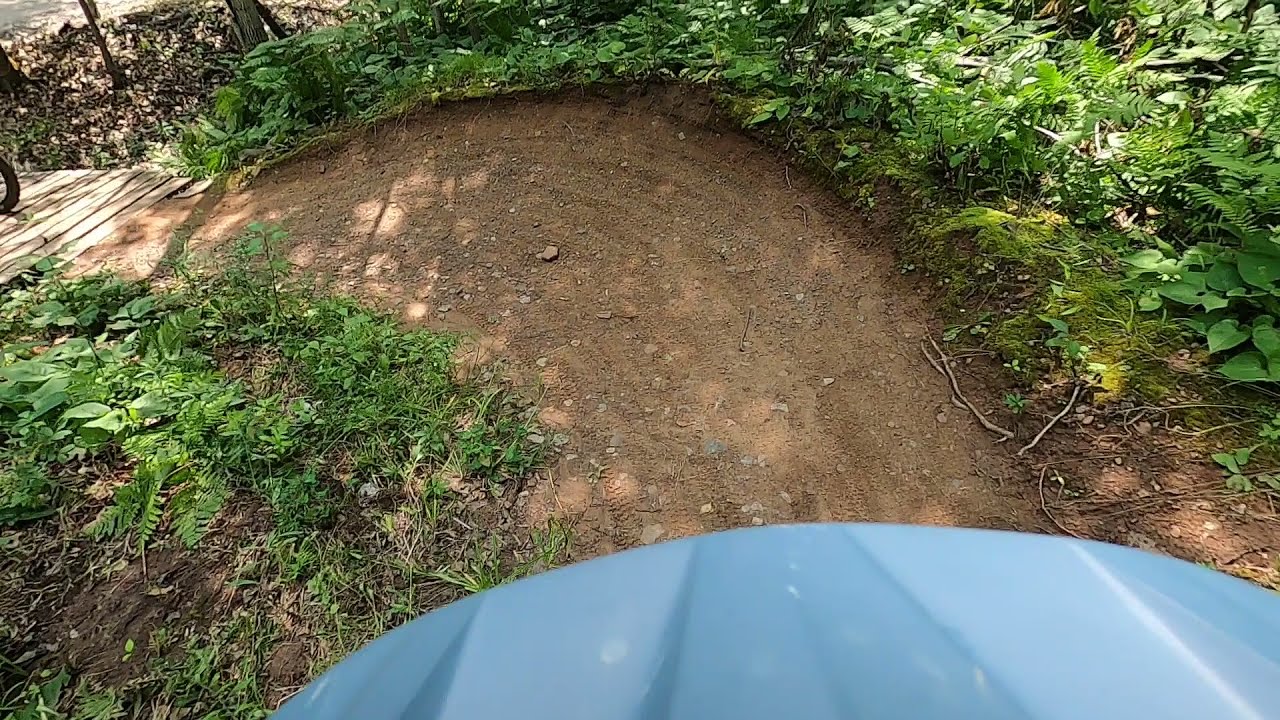The image portrays an outdoor scene, likely taken from the perspective of a bike or a motorbike. Over the hood of what looks like a blue bike fender, the dirt trail extends narrowly, bordered by green grass, ivy, ferns, and moss. The trail, marked with bike tire tracks and small stones, appears to cross over at least two wooden planks resembling a bridge, possibly constructed to span a small stream. Sunlight filters through the leaves, casting dappled light on the ground. In the upper left corner, a partially visible bicycle tire crosses the bridge, adding to the impression of a trail within a forest, surrounded by lush vegetation.